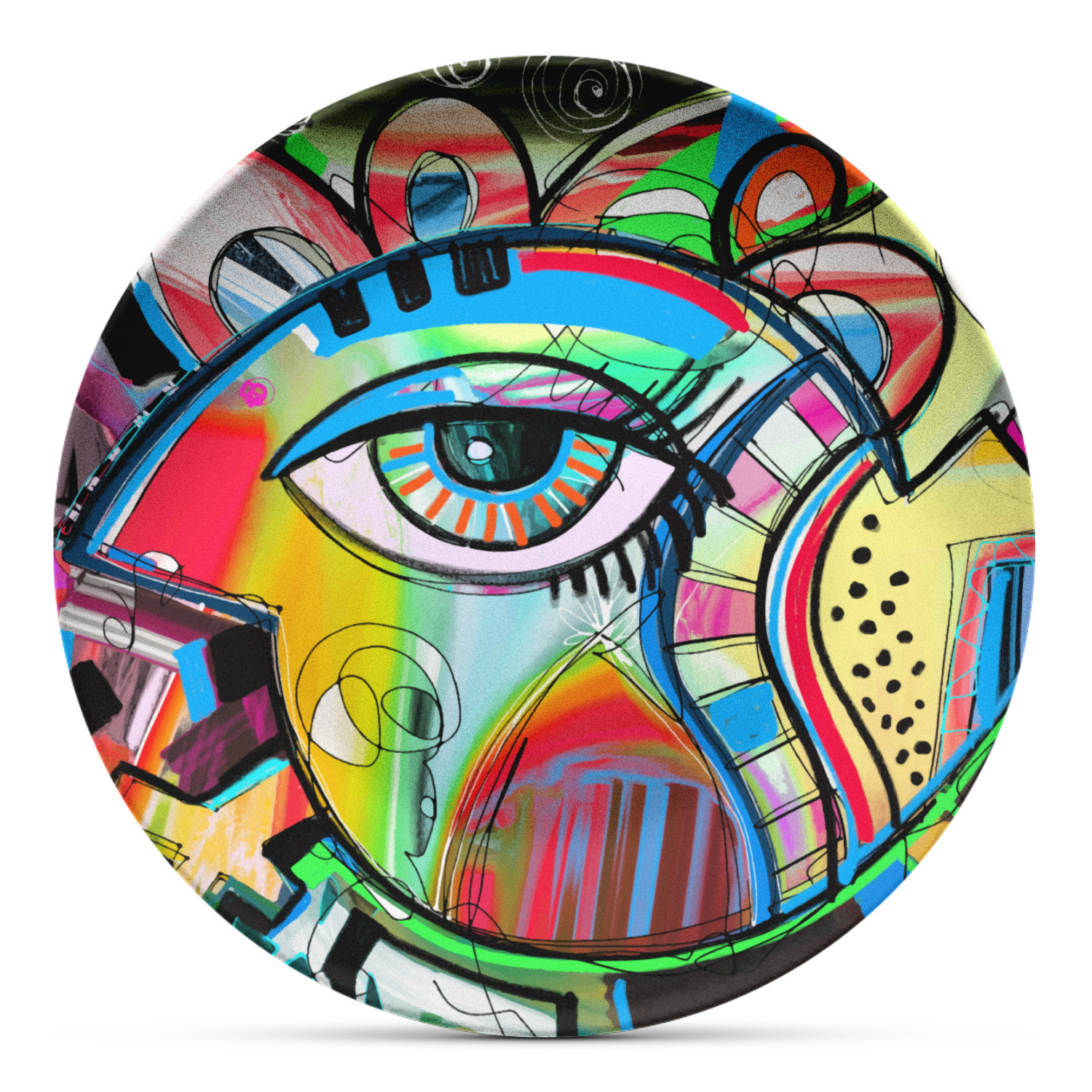The image is a detailed photograph of an artistic plate, standing upright against a stark, white background that gives it the illusion of floating in an empty void. The plate is circular, with its shadow visible at the bottom, grounding the object in the image. The entire surface of the plate is covered in an intricate, abstract painting reminiscent of modern art styles such as those by Picasso. 

The focal point of the artwork is a large, singular eye located in the center. This eye features a green iris with a black pupil, surrounded by orange lines radiating inward. The eyelid is adorned with thick, vibrant colors including blue, purple, green, and yellow, all bordered by a distinct black outline. The whites of the eye are also visible, adding to the piercing nature of the gaze.

Surrounding the eye are various geometric shapes and abstract patterns in a riot of colors, including red, black, blue, purple, and green. At the top of the plate, red and black ribbon-like shapes intermingle with white swirls. The bottom section is decorated with more obscure, tangled black lines and patterns. Collectively, the shapes and colors seem to suggest the side profile of a stylized human head, contributing to the plate's mesmerizing and complex visual appeal.